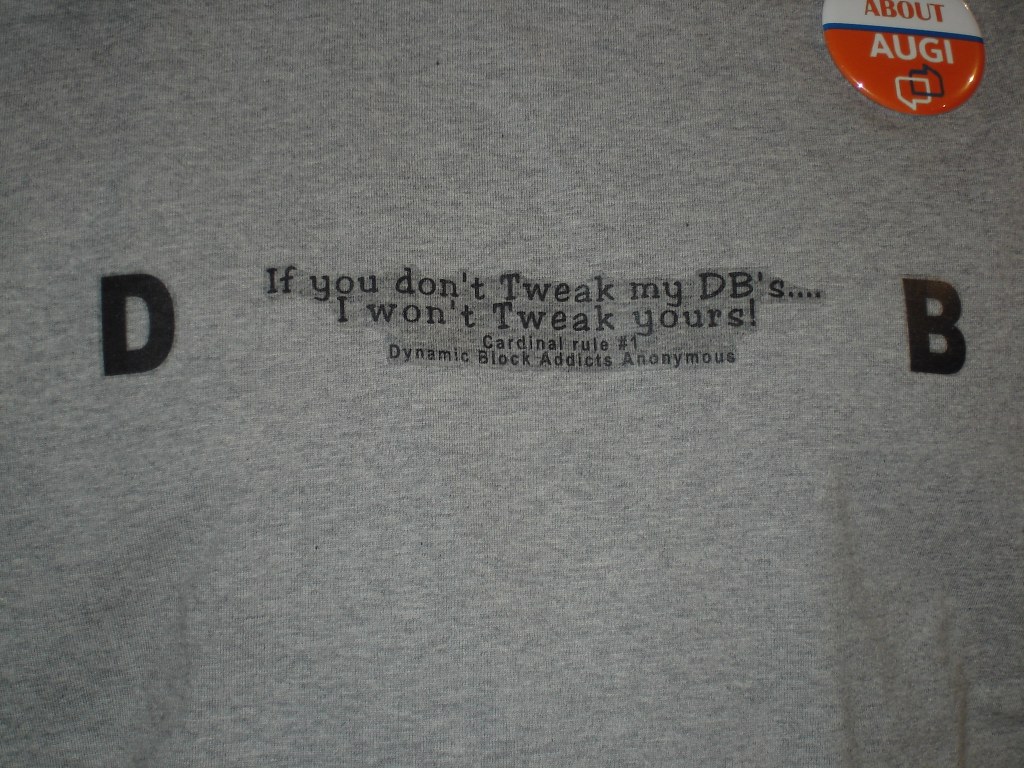A close-up image captures the details on a gray, cotton t-shirt. The entire background is filled with the soft texture of the gray fabric. Central to the image is bold black text: the letter "D" on the left and the letter "B" on the right. Between these prominent letters, less bold black text reads: "If you don't tweak my DB's..., I won't tweak yours. Cardinal rule number one, dynamic block addicts anonymous." 

In the upper right corner, a colorful button, akin to a pin someone might wear on a shirt, stands out. The top half of the button is white with red lettering that spells "about." A thin blue line separates the top from the bottom half, which is red with "AUGI" in white font. Beneath the text, small speech bubbles form a distinctive logo, adding to the button's intricate design.